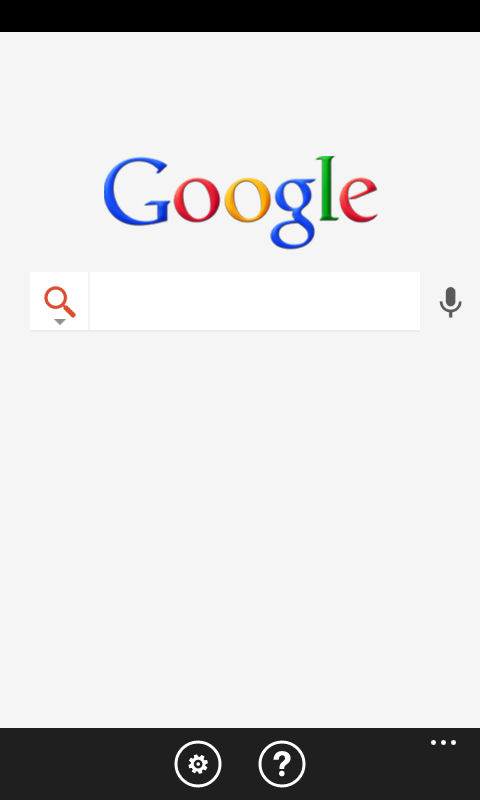A screenshot taken from a cell phone display, predominantly showcasing a whitish-gray background with thin black rectangular bars at the top and bottom edges. The top bar is narrow, stretching across the screen, while the bottom bar is slightly thicker and also spans from left to right. The bottom bar contains clickable areas: a white flower icon, a white question mark icon, and at the very left end, three horizontal white dots for additional options. Centrally, the well-known Google logo is displayed, featuring a capital 'G' in blue, followed by lowercase letters: 'o' in red, 'o' in yellow, 'g' in blue, 'l' in green, and 'e' in red. Directly beneath the logo, there is a typical Google search bar with a red magnifying glass icon on the left, an empty white text box in the center, and a microphone icon on the far right, indicating that voice input is available.